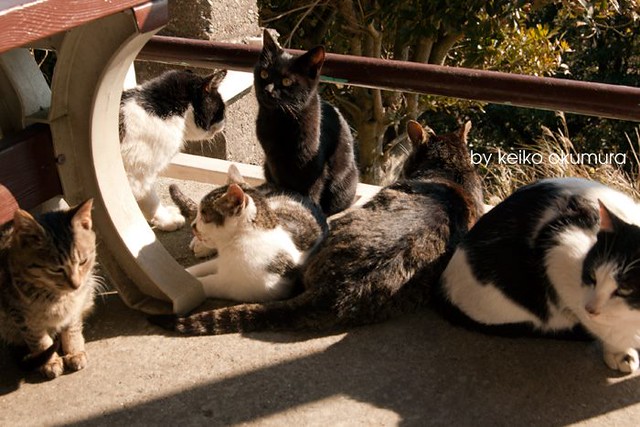A charming scene captures a group of six cats lounging and sunbathing on what appears to be a cement balcony or patio. The cats exhibit a variety of colors and patterns: two black and white, two solid black, one gray tabby, and one brown and white. They are comfortably spread out near a bench or table, with its curved leg partially visible. In the background, a brown metal railing runs horizontally and slightly diagonally across the image, adding depth to the cozy outdoor setting. The surroundings feature lush trees and grass, contributing to the serene atmosphere. The sunlight casts gentle shadows of the cats on the concrete surface, highlighting their relaxed postures. The photograph is signed in white letters with "by Keiko Okumura" in the corner.